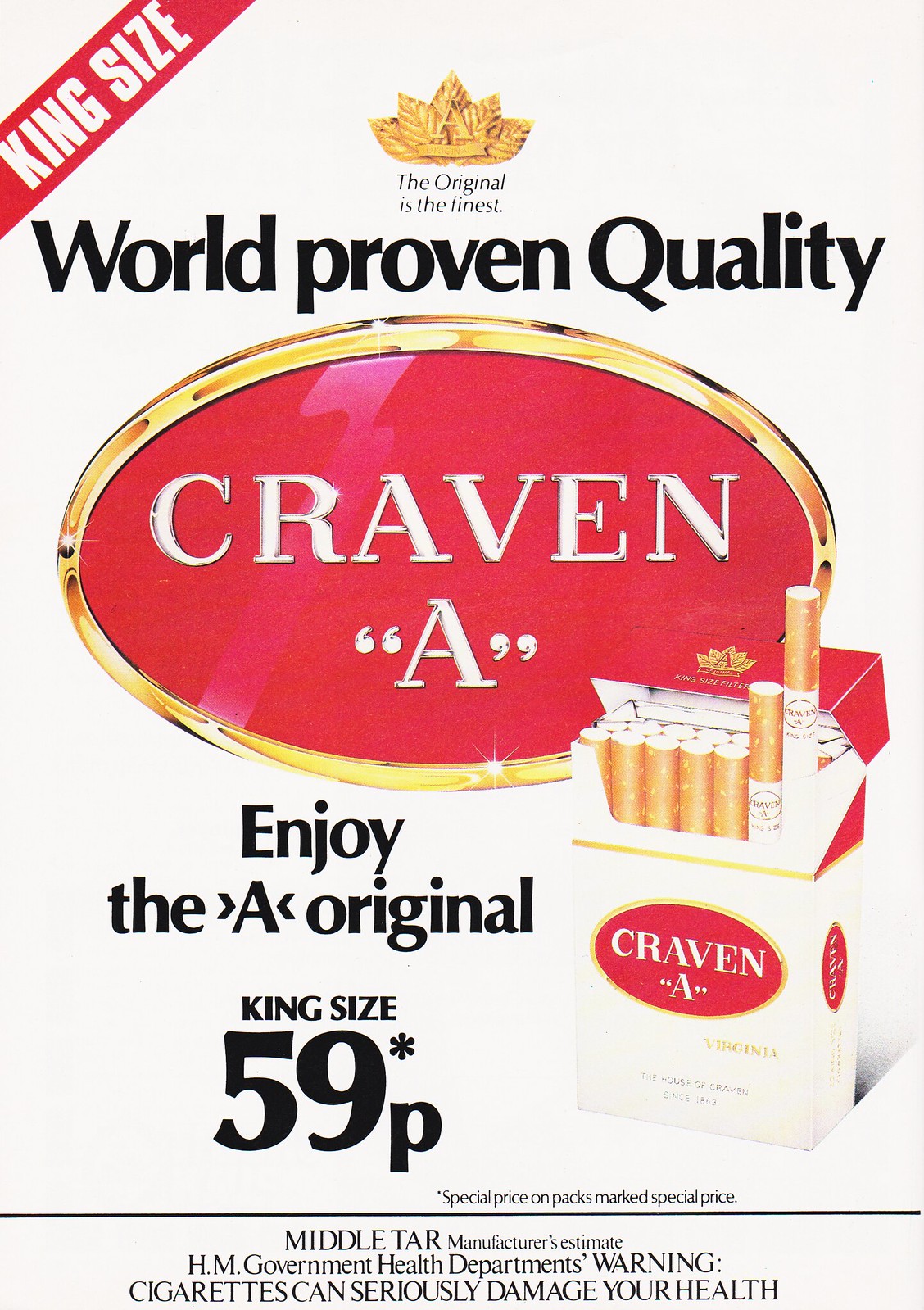This image is a detailed color photograph of a full-page magazine advertisement for Craven A cigarettes. The ad features a clean white background adorned with various black and red texts. In the top-left corner, there is a diagonal red rectangle with white text that reads "King Size." Just beneath this, a golden tobacco leaf logo is displayed, accompanied by the slogan "The Original is the Finest." Larger black text underneath proclaims "World-Proven Quality." At the center, dominating the ad, is a polished, shiny red oval with a gold border and silver lettering that reads "Craven 'A'," with the 'A' in quotation marks. To the left, a smaller black text reads "Enjoy the 'A' Original, King Size 59P." Completing the advertisement, there is an image of an open box of Craven A cigarettes with two cigarettes sticking out. The pack additionally features text that reads, "Craven A, Virginia, the House of Craven since 1863," and a health warning stating, "Cigarettes can seriously damage your health." This meticulous composition echoes both the heritage and the quality claims of Craven A cigarettes.